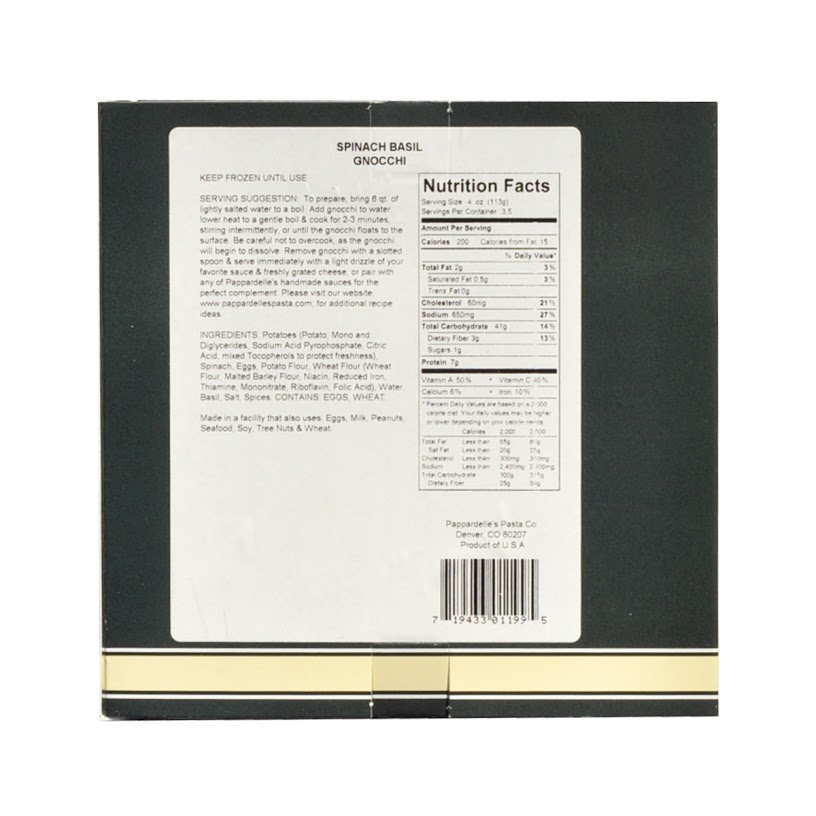This image shows the back label of a package for Spinach Basil Gnocchi on a black background. The label itself is a large white rectangle with "Spinach Basil Gnocchi" centered at the top in black print. On the left side of the label, there is a section of text providing cooking instructions, starting with "keep frozen until use." It suggests bringing six quarts of lightly salted water to a boil, adding the gnocchi, and cooking for two to three minutes, stirring intermittently until the gnocchi floats to the surface while cautioning against overcooking. This section becomes too blurry to read further. To the right of these instructions, there's a black-outlined rectangle labeled "Nutrition Facts" at the top, detailing the nutritional information including 200 calories per serving with specific breakdowns of fat, cholesterol, sodium, carbohydrates, and proteins. A barcode is located in the bottom right-hand corner of the label. The bottom of the image displays a pattern of alternating horizontal lines: starting with a strip of white, followed by a strip of black, a thick line of pale yellow, another strip of black, and ending with another white strip.